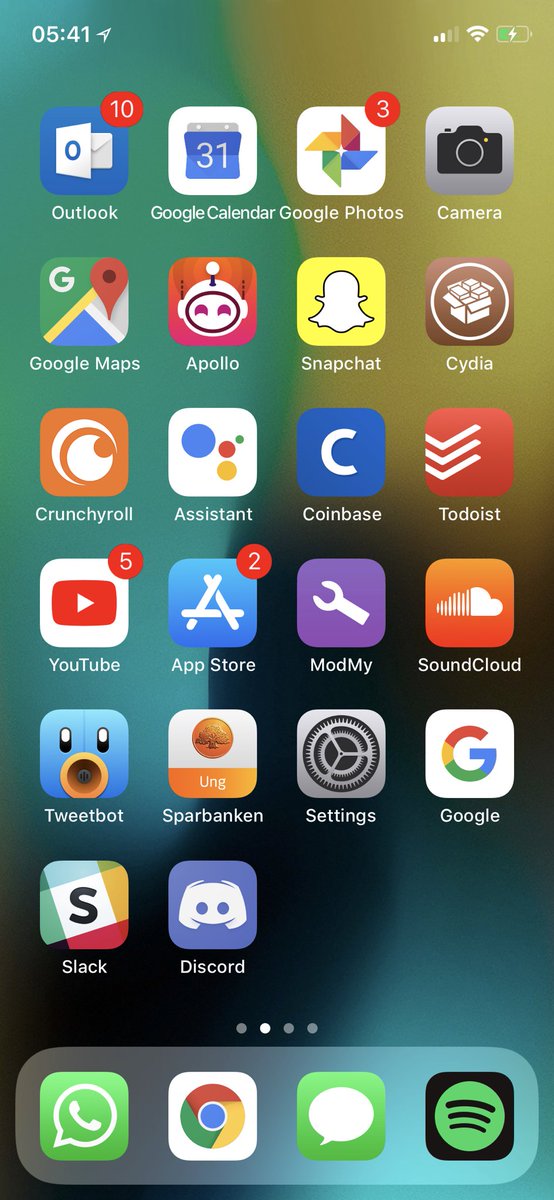This screenshot captures a portion of a smartphone's home screen. In the top-left corner, the time is displayed as 05:41, accompanied by a forward arrow, with no AM or PM indicator. On the right-hand side, the status bar reveals various connectivity indicators: a cell phone signal showing two of its four bars, a fully connected Wi-Fi signal, and a battery icon that is halfway full with a lightning bolt indicating it’s charging.

Below this, a series of app icons are arranged in a grid. The first app, Outlook, is depicted with a dark blue icon featuring an envelope and a piece of paper marked by a small blue circle. A red notification badge with the number 10 appears in the top-right corner, indicating ten new emails. Next is Google Calendar, represented by a white circle with a blue square containing the number 31, also set against a grey bezel. Following this, a multicolored pinwheel symbolizes Google Photos, complete with a red notification circle bearing the number 3.

Additional icons include:
- A dark grey square with a black camera icon, presumably for the Camera app.
- Google Maps.
- Apollo, displaying an alien with red eyes against a red and orange background.
- The Snapchat logo featuring a ghost on a yellow background.
- Cydia, shown as a white cardboard box inside a white circle over an off-brown background.
- Crunchyroll.
- Assistant.
- Coinbase.
- Totalist.
- YouTube.
- App Store.
- ModMy.
- SoundCloud.
- TweetBot.
- SPAR.
- VANKE.
- Settings, represented by a set of gears.
- Google.
- Slack.
- Discord.

The bottom bezel, which appears semi-transparent, includes additional apps: a green square with a phone icon for calling, Google Chrome, and the Messages app, displayed as a green icon with a white message bubble. Lastly, there is the Spotify icon, a black square with a green circle containing three black lines.